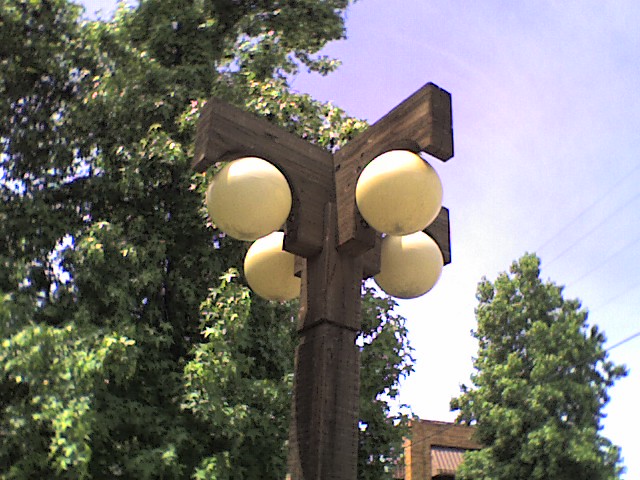The colour photograph captures a rustic, old-style wooden street lamp with a square, dark oak vertical post, viewed from a 45-degree upward angle against a vivid sky. The lamp's wooden post extends into a cross shape, with arms pointing in the 12, 3, 6, and 9 o'clock directions. Suspended from each arm is a spherical, cream-colored globe, likely made of plastic or glass, housing a light bulb within. The globes appear somewhat discolored, adding to the fixture's rustic charm.

Surrounding the lamp, on the left stands an incredibly tall tree with verdant green foliage, while a smaller tree can be seen on the right. The sky above is a striking tapestry of rich, purple-blue hues transitioning to an overexposed white near the bottom. In the bottom right corner of the frame, part of a brick building with a red and white striped awning is visible, alongside black power lines running across the scene. The overall setting exudes an outdoor, serene atmosphere on a bright, sunny day.